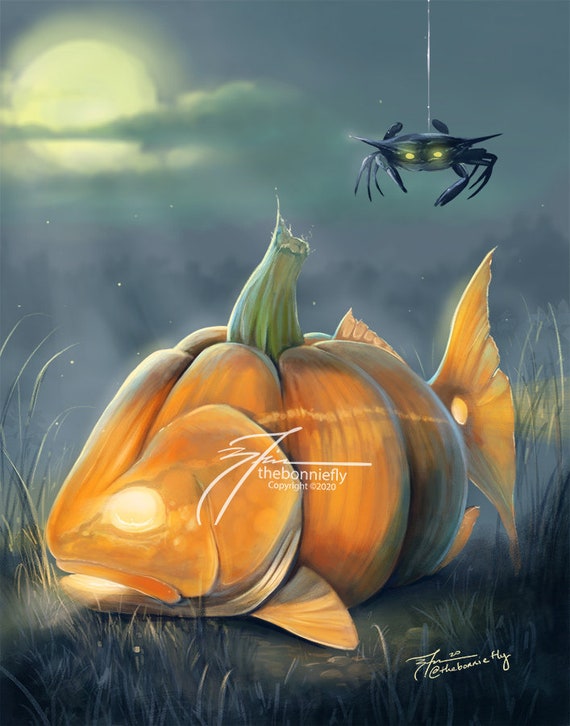This is a piece of digital art rendered as a vertically-oriented card featuring a Halloween-themed centerpiece. At the heart of the image is a jack-o'-lantern that takes the form of a fish. This unique pumpkin-fish hybrid exhibits a glowing fish face on its left side, complete with an illuminated eye and an open mouth emitting light. The pumpkin stem cleverly serves as a dorsal fin, while additional fins protrude from the bottom and toward the back, culminating in a long tail fin that also glows.

Descending from the upper right edge of the card is a spider-crab hybrid, dangling from a white thread. This creature is black with two glowing yellow eyes, leaning more towards a crab in its appearance despite its descent from a web. The background sets a spooky atmosphere with a fully-lit moon occupying the top left corner, shrouded by gray and bluish clouds against a similarly colored sky. There are hints of trees in dark hues and clusters of white stars scattered throughout.

The enigmatic pumpkin-fish sits amidst green and yellow grass, which frames the lower section of the image. Both the center of the card and its lower right corner bear a signature and text in white, citing the artist and copyright details: potentially "M fin" or "3 fin," "The Bony Fly," and "© 2020." This signature detail, written over the pumpkin, adds a final touch to the enchanting and eerie illustration.